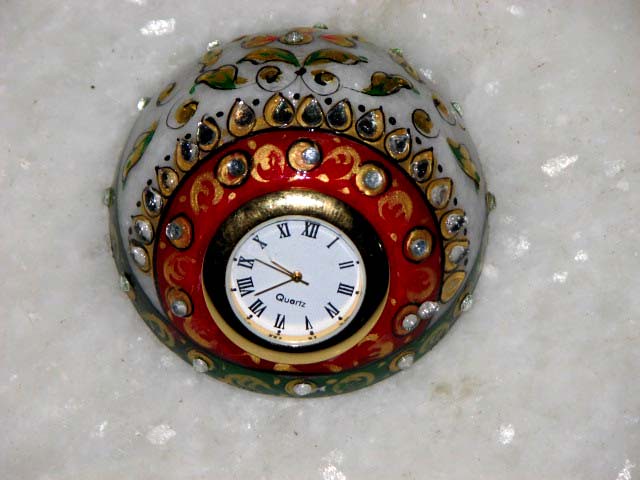The image features a spherical clock, partially encased in what appears to be ice, lending it an unusual, frozen-in-time appearance. The clock is dirt-streaked, suggesting it may have been exposed to outdoor elements. The clock's distinctive spherical design is adorned with multiple intricate layers. At its core, the clock face features Roman numerals and bears the inscription "Quartz." Surrounding the clock face is a gold rim, followed by a red circular band punctuated with dots. Outside this, a white section decorated with leaf patterns and various other designs completes the elaborate outer layer.